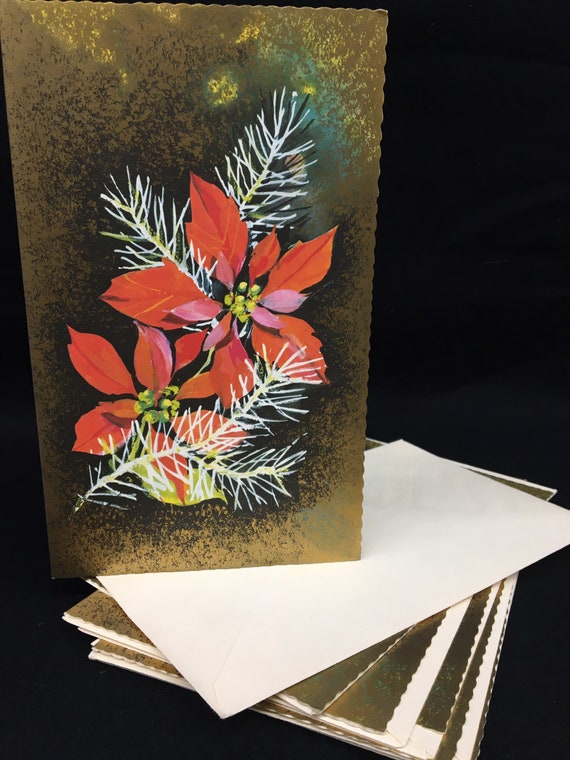This photograph depicts a collection of Christmas cards arranged on a black background. Most of the cards are lying flat, forming a pile under a single, prominently displayed card that stands atop a white envelope. The standing card features a striking design with a dark, metallic gold background that shimmers in places. Its focal point is a pair of vibrant red poinsettia flowers, each adorned with clusters of small green buds at the center. White, spiky twigs encircle the blooms, with some branches positioned in front of and some behind the leaves, adding depth to the composition. The card's ornate details are complemented by splotches of brown and yellow, enhancing its festive appearance.